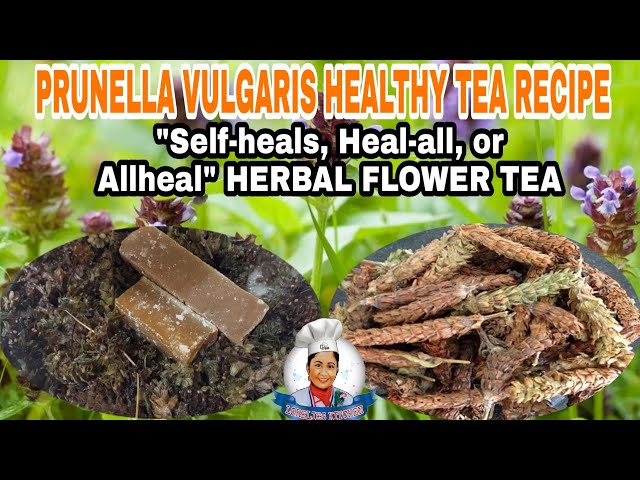The YouTube thumbnail features Camilla O'Briell promoting a Prunella vulgaris healthy tea recipe, also known as "self heals" or "all heal" herbal flower tea. The background showcases a tall, purple flower, presumably the Prunella vulgaris plant. The thumbnail displays two close-up dishes: the one on the left contains two dark brown bars lying on a bed of green and brown herbs, possibly representing processed or dried tea form. The right dish shows dried, cob-like tips of herbs, appearing as if freshly picked and dried. In the bottom center, there is an image of a woman wearing a chef’s hat, possibly of Indian or Middle Eastern descent, which adds a culinary touch to the presentation.